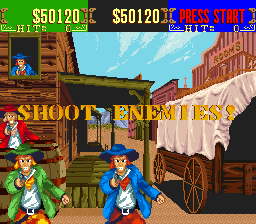This detailed caption effectively describes the screenshot from the video game:

In this small, square screenshot from a computer game, a classic Western scene unfolds. On the right-hand side, there's an intricately detailed wagon featuring a white cover, brown wheels, and a brown body. Behind the wagon stands a building labeled "Rooms," suggesting it functions as a hotel. To the left, a saloon captures attention with its inviting facade. 

In front of the saloon, three distinct outlaws are poised for action. The first outlaw sports a blue jacket and matching blue hat, while the second outlaw is dressed in a green jacket with a corresponding green hat. Behind them stands a third outlaw donning a red jacket and red hat. Each of these menacing figures brandishes a firearm, all aimed directly at the viewer, amplifying the tension of the scene. 

At the center of the screen, the text "Shoot enemies" serves as a clear directive. The upper 10% of the screen is dedicated to various scores. On the left, in yellow lettering, it prominently displays "$50,120." Beside it, in a different format with yellow text on a black background, the same amount "$50,120" is repeated. To the right, a blue section with red letters stands out, instructing players to "Press Start." This screenshot vividly captures the thrilling and dangerous atmosphere of the game's Western setting.